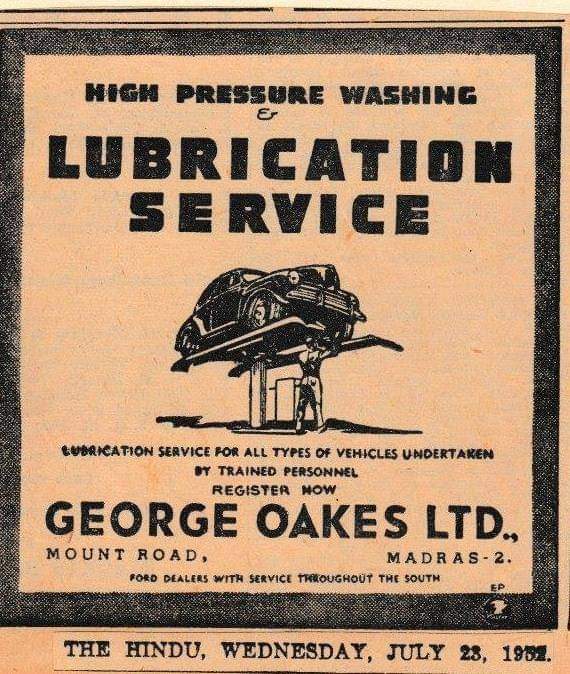This sepia-toned advertisement poster with a black border features an old-school business promotion for George Oaks Limited, located on Mount Road, Madras 2. At the top of the poster, bold black text announces "High-Pressure Washing and Lubrication Service," with "Lubrication Service" prominently displayed in larger, bold letters. Below this headline, a black outlined, animated image shows a mechanic working underneath a car, possibly a Volkswagen Beetle, lifted on a riser. The text beneath the image reads: "Lubrication service for all types of vehicles undertaken by trained personnel. Register now." The poster also notes the expansive reach of the service, mentioning, "Four dealers with service throughout the South." At the bottom, the poster specifies the source, "The Hindu," and the date, which reads "Wednesday, July 25th, 19—," though the year is smudged and possibly says either 1932 or 1957.